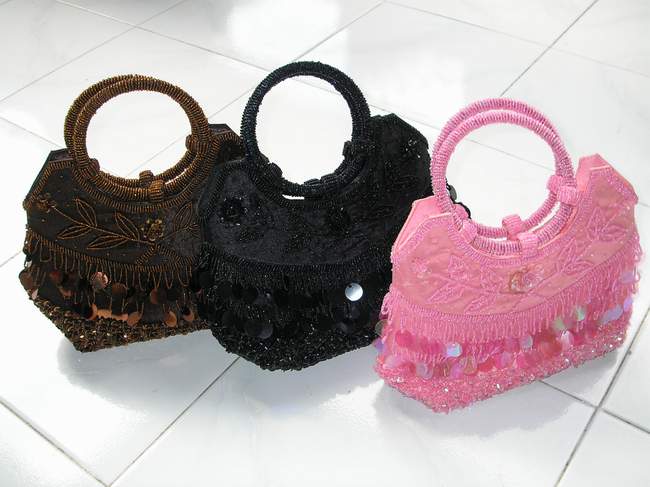In this amateur photo, we are looking down on a white tiled floor illuminated by a light that causes the three purses to reflect slightly on the surface. The rectangular image, oriented horizontally, showcases three identical handbags arranged from left to right: a dark copper, golden brown bag, a black bag, and a pink bag. Each handbag features distinct circular wicker handles attached to a rounded top. They are adorned with an embroidered floral pattern on the upper section, and the lower part is embellished with hanging tassels, beads, and potentially large sequin-like decorations. Despite their intricate detailing, the purses do not appear to be of high quality.